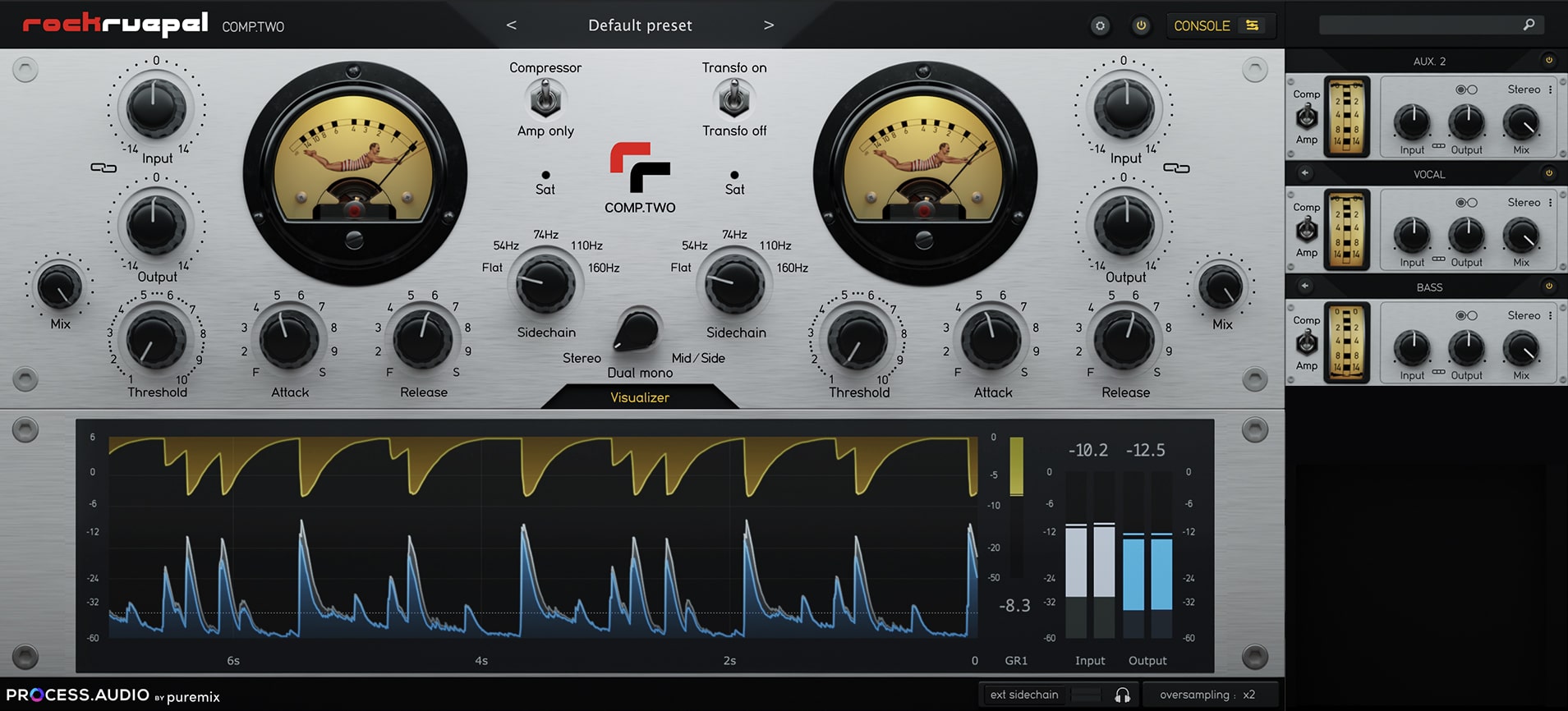This image depicts a detailed and sophisticated audio soundboard, likely a digital music studio interface or a digitized analog device. The console, mostly white with numerous black knobs, features black dials arranged in an L-shape to the left and a backward L-shape to the right, with two prominent larger dials positioned centrally. These prominent dials display a man in a bathing suit, suggestive of a vintage design or analog homage. 

The screen towards the bottom showcases spiky blue and gold sound waves, indicative of an active audio monitoring system. Various text labels include "Rock Rue Pell Console" at the top and "process.audio" or "pure mix" at the bottom. The middle section reads "default preset,” while other labels such as "exl sidechain," "oversampling x2," and "compressor" are situated on the right side, where smaller racks of devices are also visible.

Additional numerical readings like "10.2" and "minus 12.5" appear alongside a gauge for input (white) and output (blue). Two blue level bars add further detail to the visual information presented by the interface, ensuring it provides comprehensive, at-a-glance data essential for audio production or management. This intricate setup hints at a blend of modern digital controls with a vintage aesthetic, possibly used in professional audio processing or specialized fields.